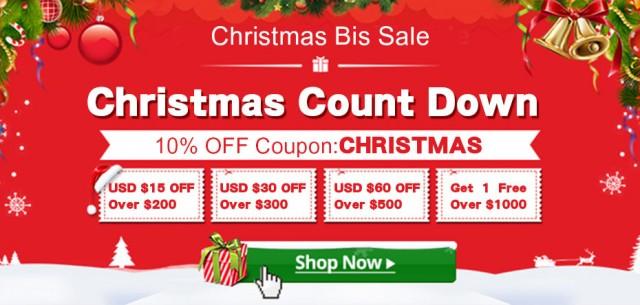This is a detailed description of a Christmas sale advertisement displayed on a computer screen:

The ad headline reads "Christmas Big Sale" in bold, festive lettering. Flanking the headline, there are decorative white lines framing a central image of a beautifully wrapped Christmas present, serving as an elegant logo. The top corners of the advertisement are adorned with holiday ornaments: on the left, red circular baubles hang amidst green foliage, while the right side features golden bells tied with a vibrant red bow.

Beneath the headline, bold white text announces a "Christmas Countdown," accentuated by a decorative ribbon below it. Printed on the ribbon is a promo code—"10% OFF COUPON: CHRISTMAS"—which customers can use at checkout to receive a 10% discount.

Further down, the ad showcases four different discount coupons:
1. USD $15 off on purchases over $200.
2. USD $30 off on purchases over $300.
3. USD $60 off on purchases over $500.
4. A special offer to get one item free with purchases over $1,000.

At the bottom of the ad, a green button with the call-to-action "Shop Now" invites users to start shopping and take advantage of the holiday deals.